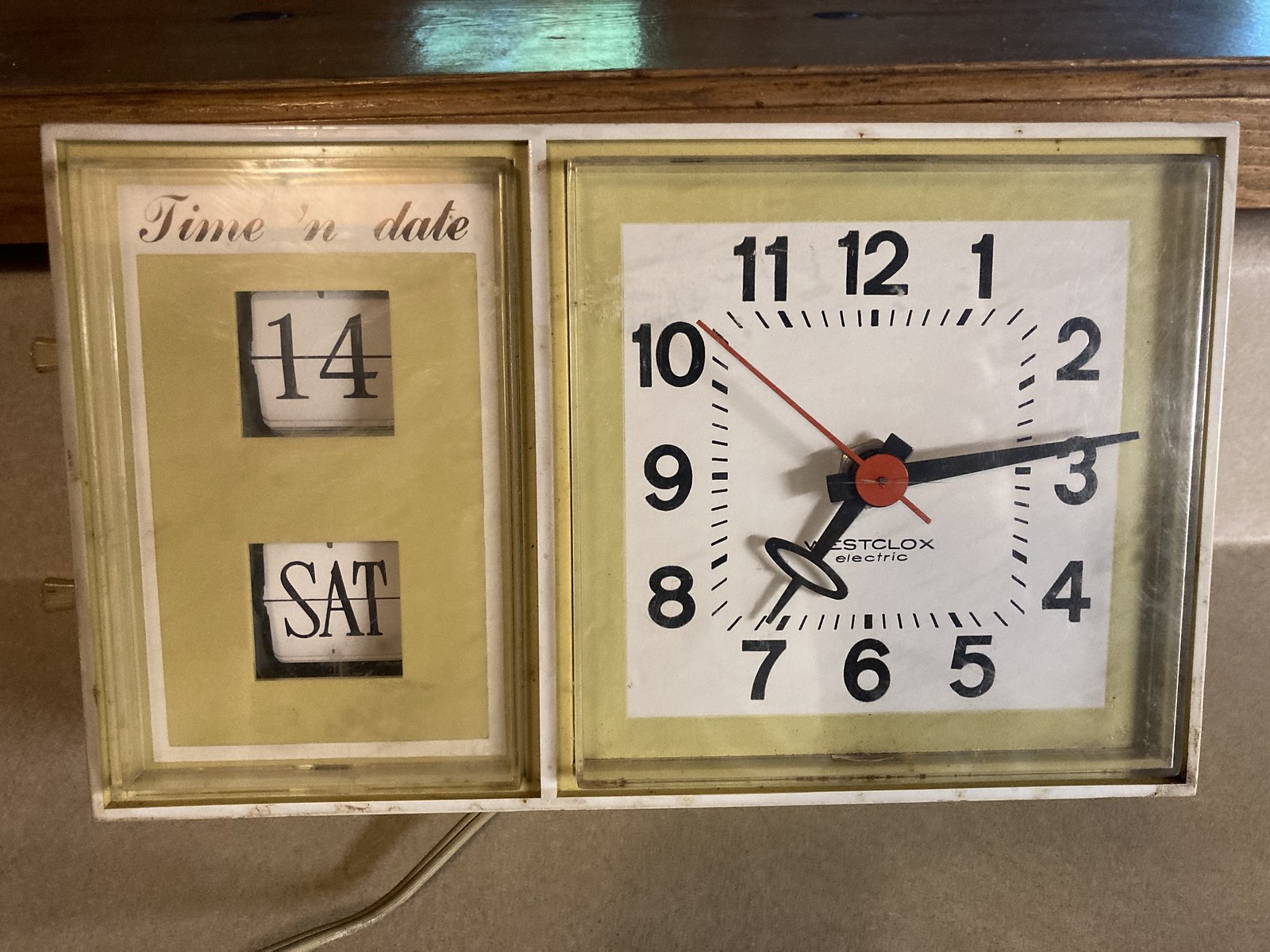This detailed photograph showcases a vintage electric Westclox clock, likely from the 1960s, placed on a gray countertop. The clock, designed for tabletop use, features a square face with a gold border and white background. Black numbers (1 through 12) are arranged around the clock face, accompanied by black hour and minute hands, and a distinct red second hand. The clock is marked with the brand name "Westclox Electric" in black font. To the left of the clock is a smaller, complementary section also framed in gold with a white background, displaying the date "14" and the day "Sat" in black font. The setup indicates the clock's functionality for both time and date display. The backdrop includes a black and brown wood frame, contrasting against a white wall, providing a warm, homely setting. An extension cord, hinting at the clock's electric nature, trails from the left side of the image. The time displayed on the clock is precisely 7:14.